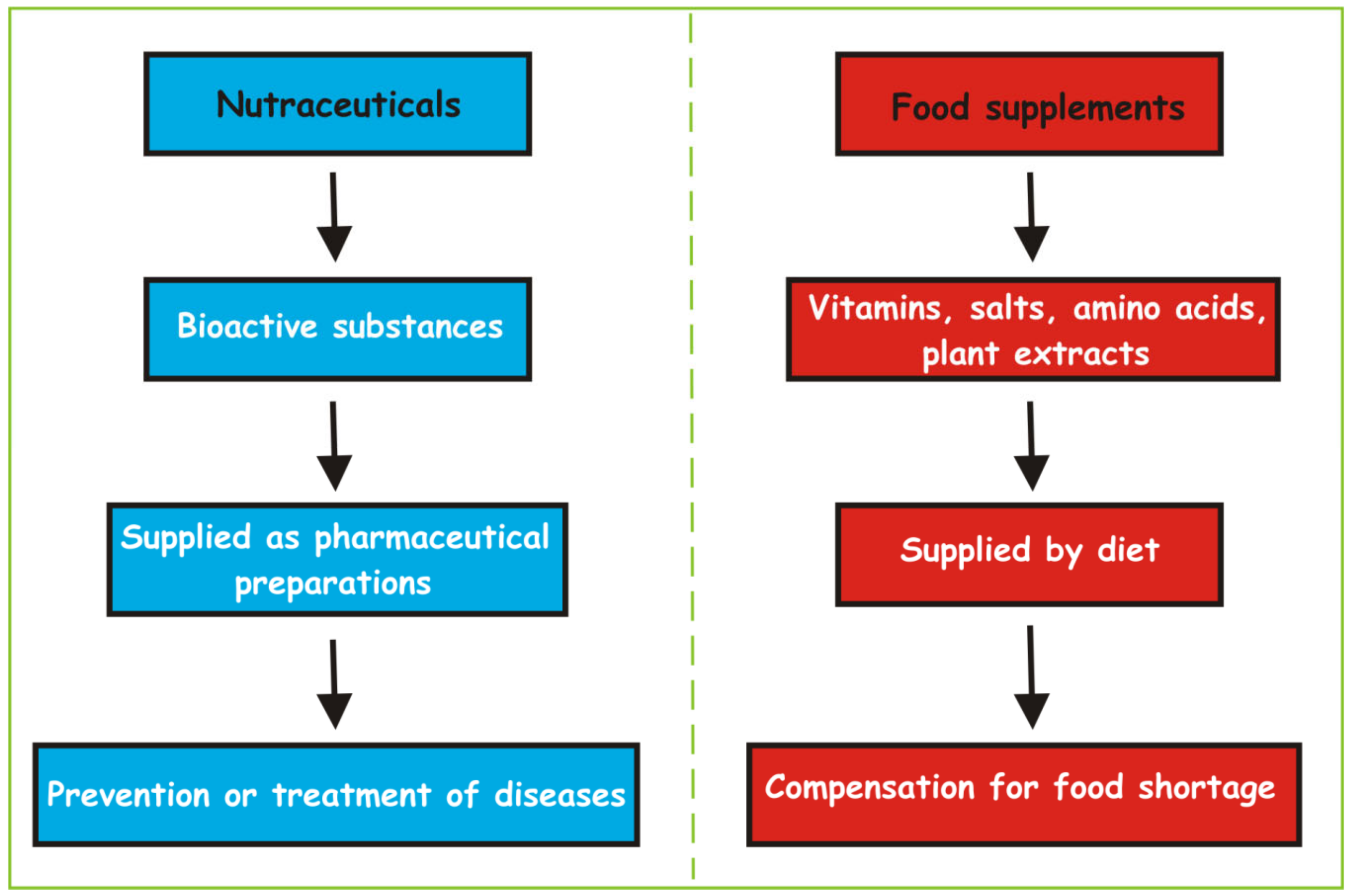The image features a detailed, digitally generated flowchart diagram with a green border and a dotted green line dividing two columns. The left column, highlighted in blue rectangles with black arrows pointing downward, details the progression starting from "Nutraceuticals," moving to "Bioactive substances," followed by "Supplied as pharmaceutical preparations," and concluding with "Prevention or treatment of diseases." The right column, consisting of red rectangles with black arrows pointing downward, begins with "Food supplements," continues to "Vitamins, salts, amino acids, plant extracts," then "Supplied by diet," and ends with "Compensation for food shortage." The text within the image is prominently in black or white. The overall style of the image is scientific, representing a comparative analysis of nutraceuticals and food supplements.